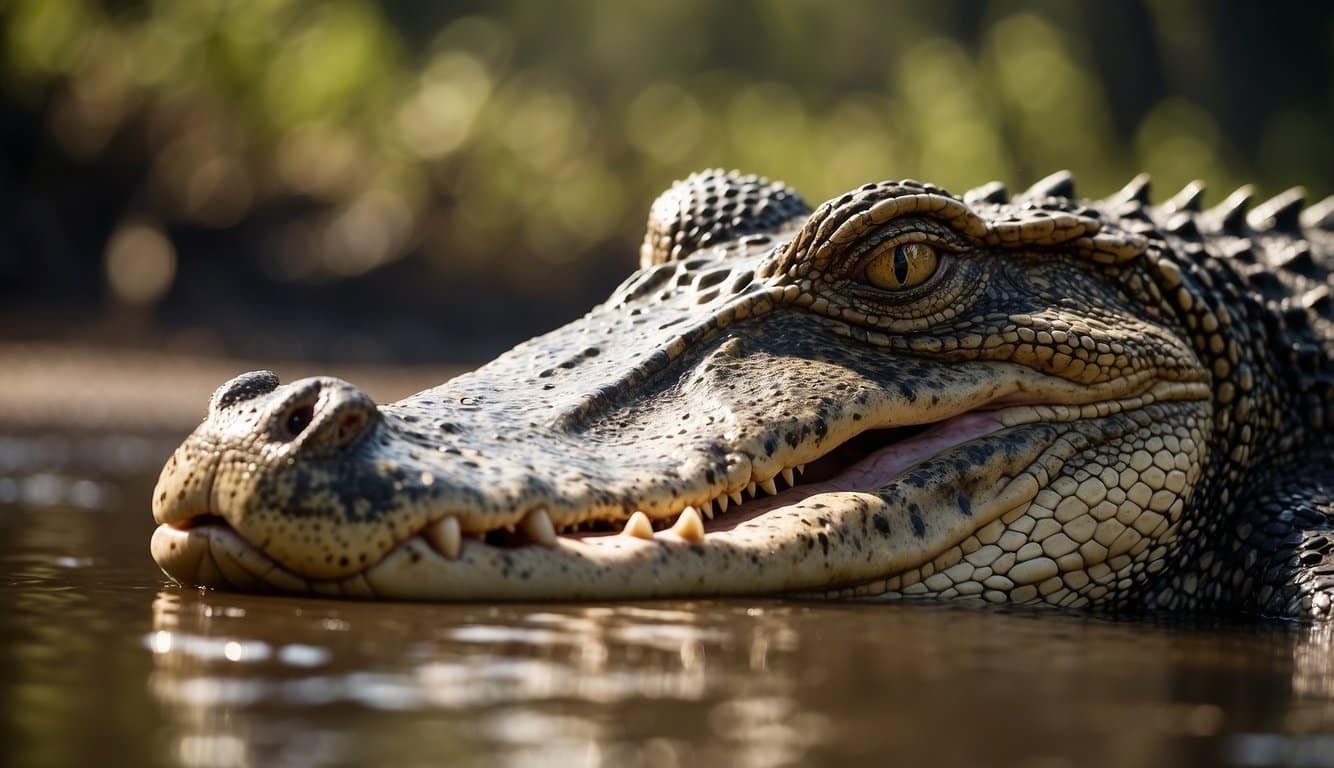The photograph captures a crocodile or alligator, barely submerged in shallow, dark, and murky water, with its long, flat snout and head prominently displayed just above the surface. The reptile's head features a distinctive dark green coloration with lighter green hues around its mouth, where a few teeth jut out from the bottom jaw, complemented by a whole row of slightly hidden teeth. Its mouth is slightly open, revealing a glimpse of pink fleshiness inside. The creature's yellow, cat-like slit eye stares directly into the camera, framed by scales around its eyes and the bulb at the back of the eye. The nose tilts slightly upward, while the spiky ridges along its back trail off into the distance towards the blurred shoreline and indistinct trees in the background. The scene is captured with professional clarity, highlighting the intricate details of the crocodile's scales and the texture of its rough, formidable skin.